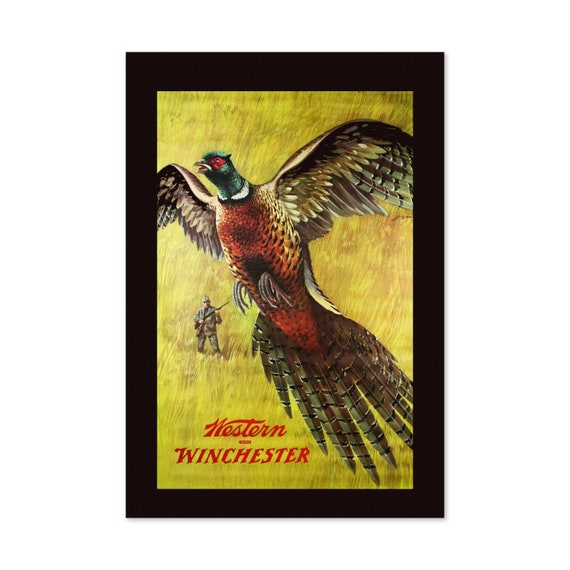This vintage advertisement poster for Winchester Rifles features a vivid, high-quality illustration by renowned artist Weimar Purcell. Dominating the composition is a striking pheasant in mid-flight, showcasing its vibrant green head, red eye, reddish-brown chest, and brown and gold feathers. The bird's magnificent wings are spread wide, and its beak is open as it flies against a predominantly yellow background, reminiscent of a cornfield or wheat field. In the distance, a male figure dressed in camouflage and a hat appears small and understated, emphasizing his intention to blend into the environment. He is holding a gun and intently watching the pheasant, poised as if preparing to shoot. At the bottom of the poster, in red text, the words "Western Winchester" are prominently displayed, further indicating its purpose as a historic advertisement for Winchester firearms.